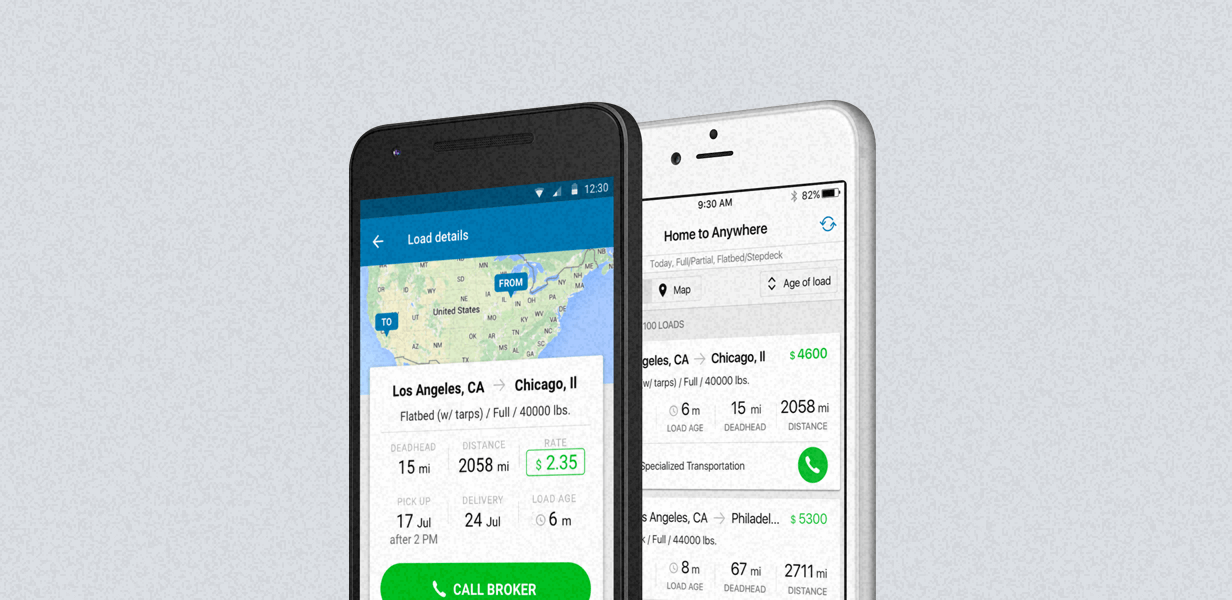This image, seemingly sourced from a website, features a graphical representation of two smartphones presented against a light gray, slightly textured background. The texture of the image could be intentionally granular. 

**First Phone (Black) Details:**  
- Positioned on the left, this black smartphone displays a detailed map highlighting a route from Los Angeles, California, to Chicago, Illinois. 
- The display includes operational details: "Flatbed with tarps, full 40,000 pounds," along with specific metrics such as:
   - Deadhead: 15 miles
   - Distance: 2,058 miles
   - Rate: $2.35 per mile
   - Pickup: 17 July after 2 p.m.
   - Delivery: 24 July
   - Load age: 6 months
- A prominent green button labeled "Call Broker" is visible.

**Second Phone (White) Details:**  
- The white phone is partially obscured beneath the black phone, leaving the far left edge out of view. 
- At the top, it displays "Home to Anywhere," accompanied by clickable options for a map and a drop-down menu focusing on "Age of Load."
- The screen shows similar details for the route from Los Angeles, California, to Chicago, Illinois, with the following metrics:
   - Rate: $4,600
   - Load age: 6 months
   - Deadhead: 15 miles
   - Distance: 2,058 miles
- A round button labeled "Specialized Transportation" is displayed.
- Below, another set of metrics is partially visible:
   - Load age: 8 months
   - Deadhead: 67 miles
   - Distance: 2,711 miles

The unidentified brand of the smartphones, their rounded corners, and the positioning of functional elements such as the microphone and flash initially suggest they might be iPhones, but the specifics are unclear from the image.